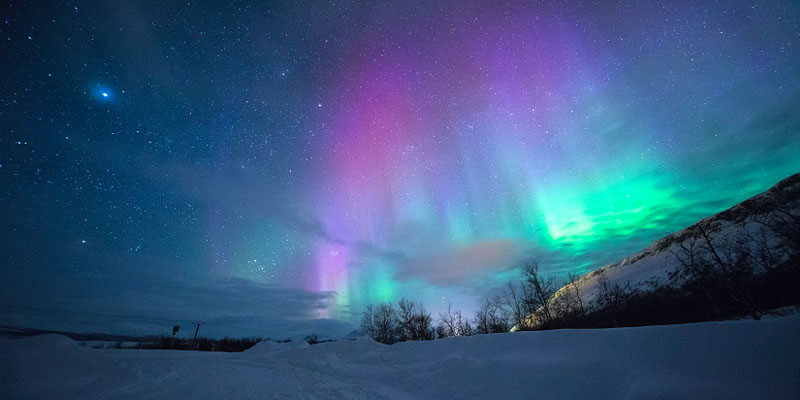This is a stunning color photograph capturing the aurora borealis, or Northern Lights, in a panoramic, wide-angle view. The scene is set on a clear winter night under a dark blue and milky sky sprinkled with numerous twinkling white and blue stars, including an especially bright star in the upper left corner, possibly with a halo or cloudy area around it. Dominating the middle and right side of the image, the aurora borealis displays vibrant and dynamic hues of purple, magenta, pink, mint, green, and neon blue, radiating down from the sky in ray-like streaks. Below this celestial spectacle, the ground is thickly covered with snow, and the image is framed by the outline of bare, dark trees. Toward the right side of the photograph, a snow-covered hill, dotted with shrubs and trees, fades off to the side, adding depth and a touch of the terrestrial landscape to the mesmerizing sky above.